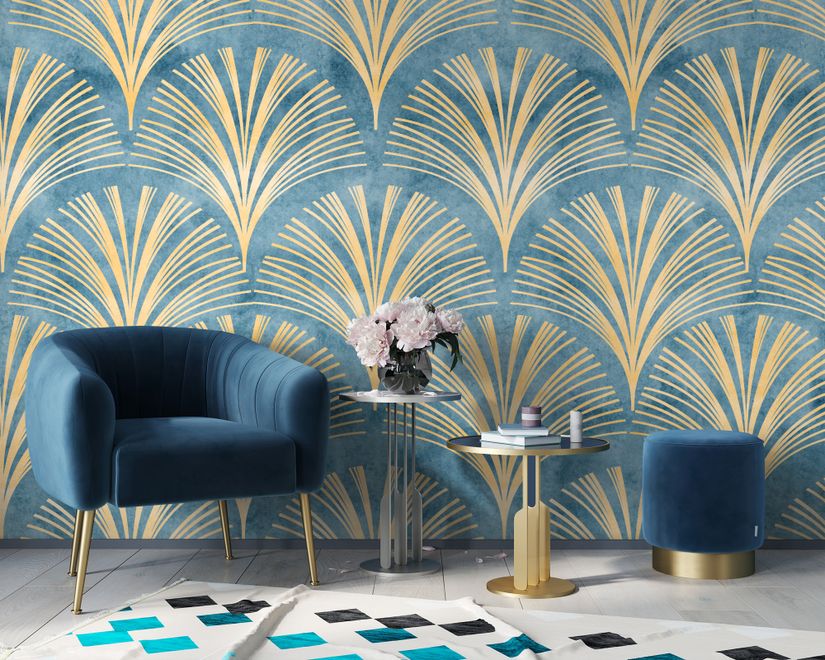The photograph showcases a stylish sitting area in a home, featuring a mix of mid-century modern and opulent accents. Against a striking wall adorned with a fan-shaped gold pattern on a slate blue background, the arrangement includes a plush, blue velvet-like chair with gold legs, exuding comfort and elegance. Adjacent to the chair is a trio of tables: a silver metal side table holding a vase with white and lightly pink flowers, a smaller gold table decorated with a couple of books and jars, and the matching blue cylindrical ottoman with a gold base that complements the chair. The entire setup rests on a light-patterned rug, meticulously detailed with diamond shapes in black, teal, and blue, set against a soft white background. The scene is unified by an undercurrent of teal and gold hues, creating a cohesive and sophisticated atmosphere.